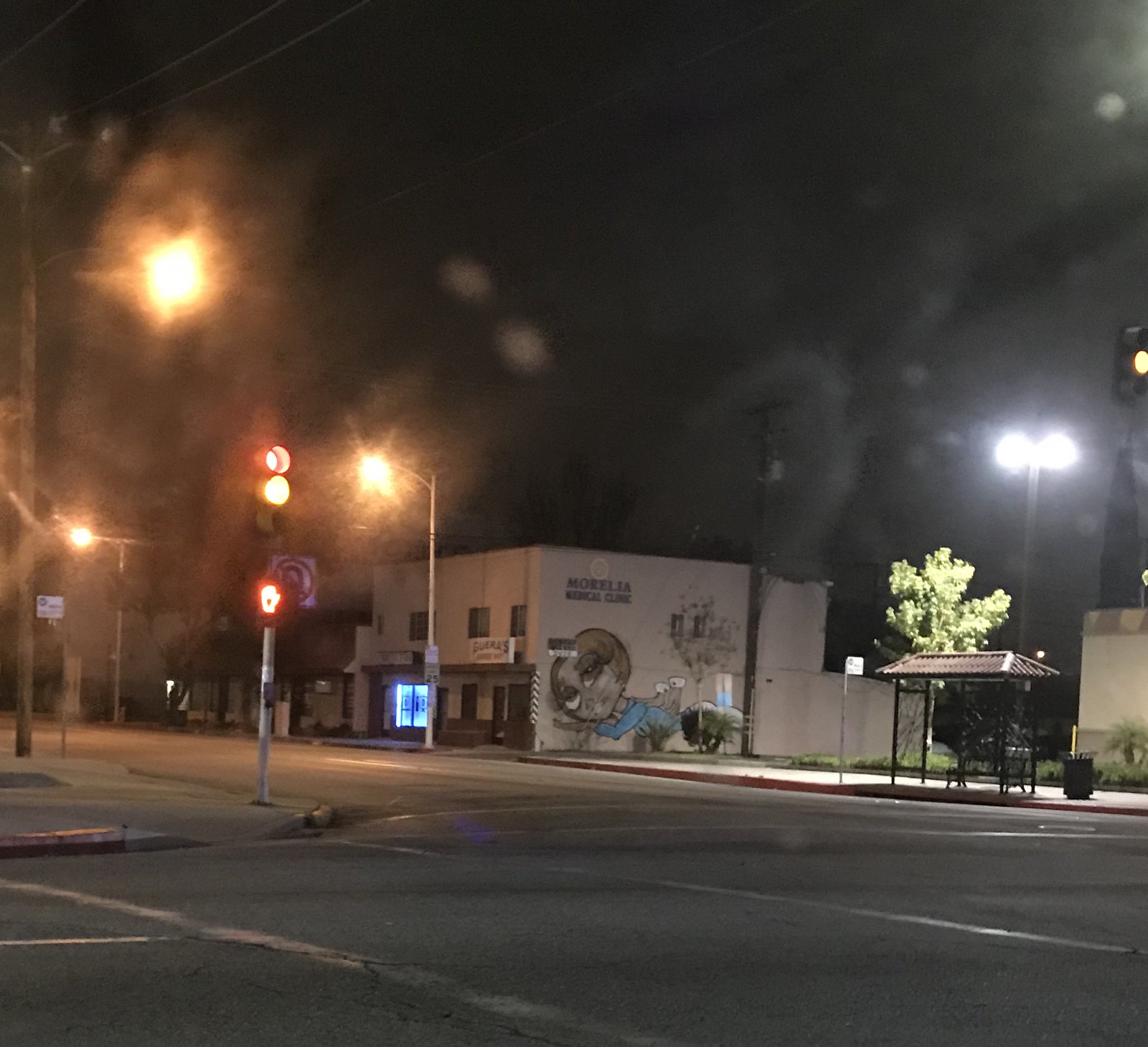This nighttime outdoor photograph captures a serene and rainy street scene. The street is devoid of cars, and the distinctive amber-hued glow from the streetlights creates a slightly blurred effect, indicating the presence of rain. Dominating the intersection is a stoplight, glowing red and yellow, accompanied by a pedestrian signal displaying a hand, warning not to cross. Across the street, a quaint bus stop with a hip-shaped tile roof and an ornate black wrought-iron design stands prominently. The bus stop features a bench and a trash can nearby. Adjacent to the bus stop is an open space leading to a square building with a flat roof. The side of this building is adorned with a vibrant mural depicting a Bratz doll character. This cartoon figure, with exaggerated eyes, long lashes, and pink lips, is in a bending pose as if about to touch the ground, while her gaze is directed upwards towards the camera.